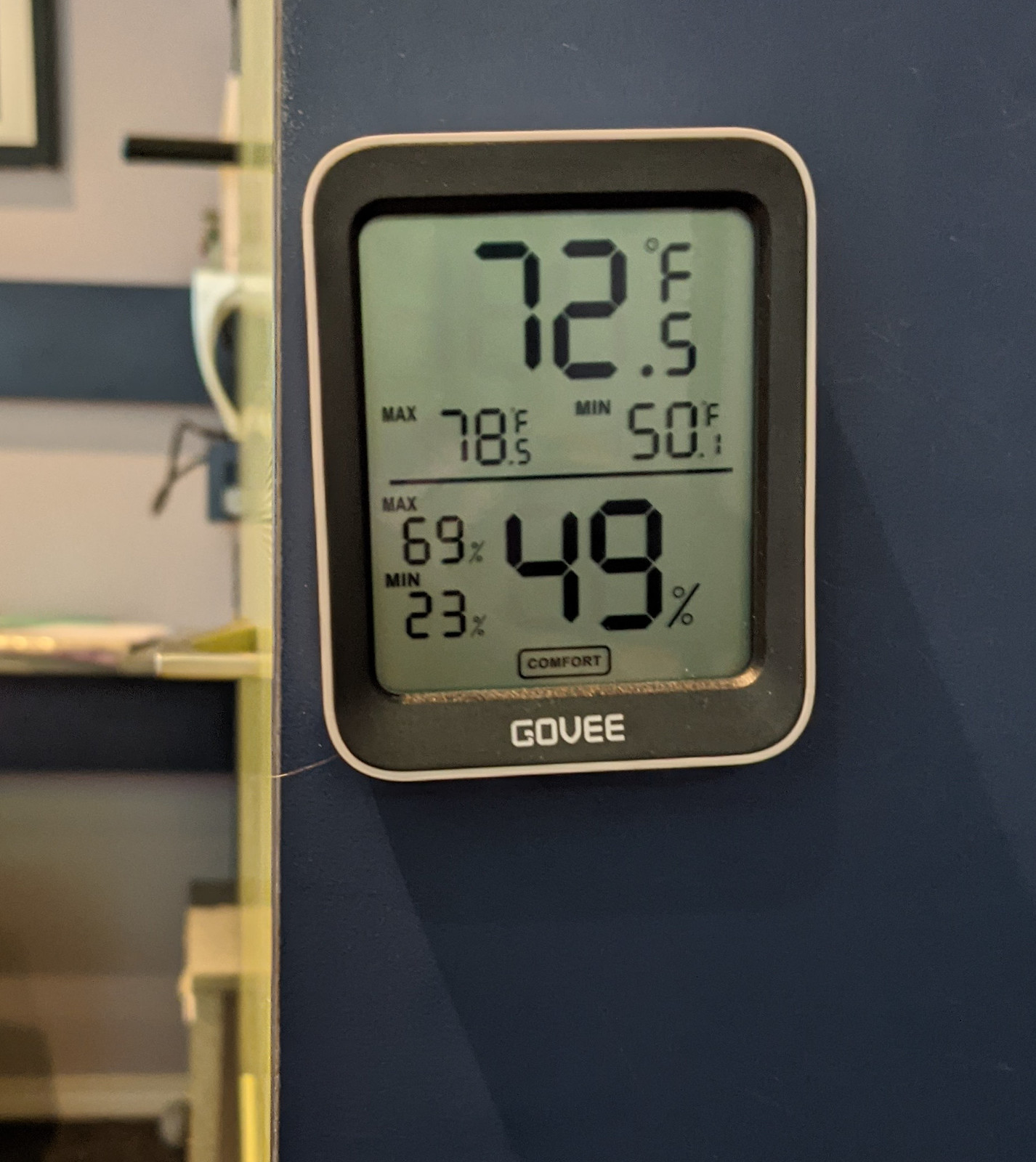This close-up image captures a digital thermometer and humidity monitor, likely a household device, mounted on a blue wall. The blue wall dominates approximately three-quarters of the image, from right to left, with the remaining quarter on the left side showcasing a blurred angle, possibly the adjoining wall. The monitoring device is a Covee model, evident from the brand name "COVEE" inscribed on the bezel surrounding the LCD display. The display itself is divided into two sections. The upper section presents the temperature readings: 72.5 degrees Fahrenheit as the current temperature, with a maximum of 78.5 degrees and a minimum of 50 degrees. The lower section shows the humidity levels: a large 49%, with a recorded maximum of 69% and a minimum of 23%. Additionally, the word "comfort" is prominently displayed beneath the current humidity reading, indicating an optimal living environment.